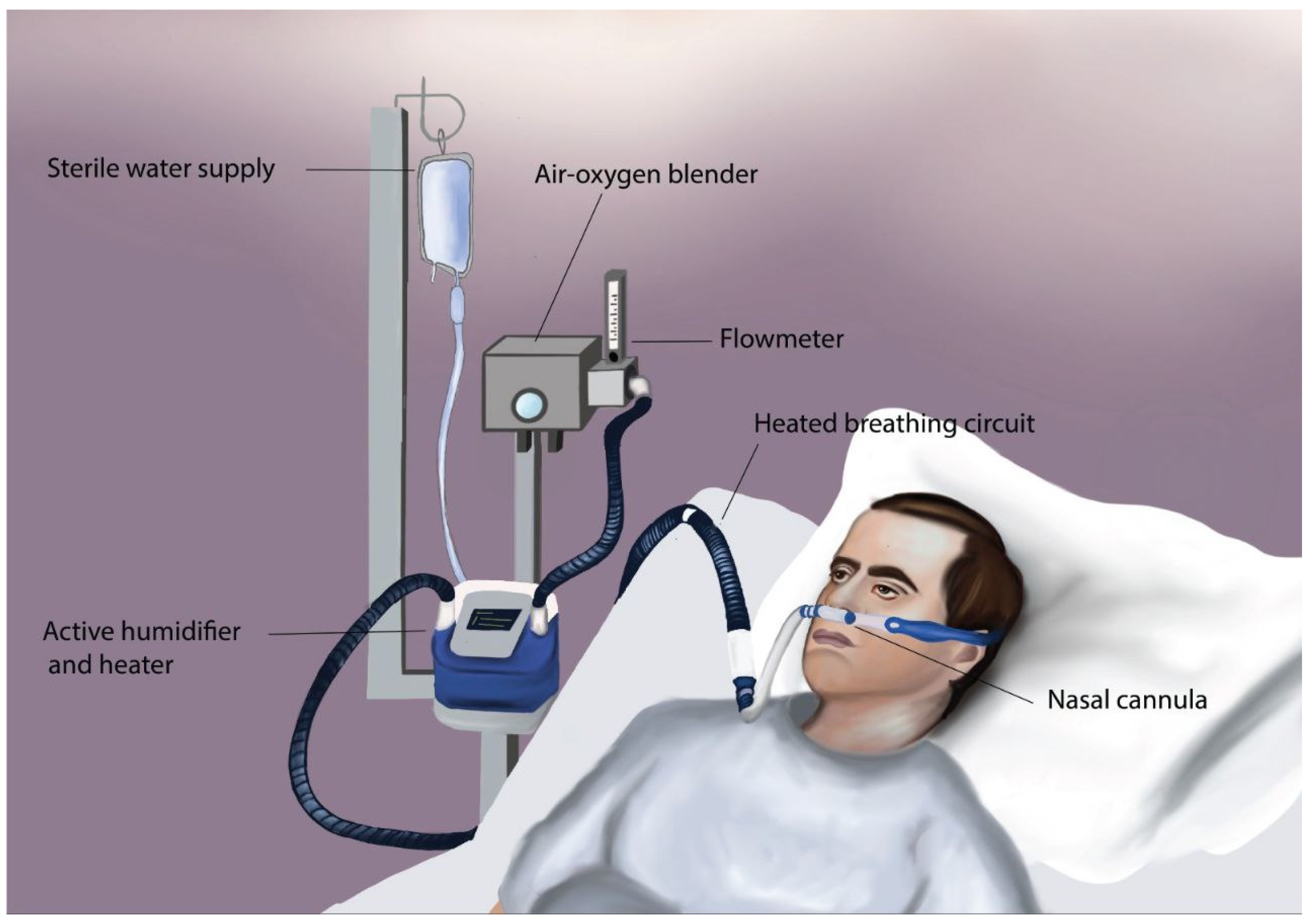The detailed medical illustration shows a male patient with short brown hair lying in a white hospital bed, resting against a white pillow. The background is a blurry lavender mauve color, giving the image a serene but clinical atmosphere. The patient appears to be receiving treatment through a complex medical apparatus positioned to the side of the bed. This device comprises an intricate assembly of tubes and machines, meticulously labeled for clarity.

Attached to the patient via a nasal cannula, the tubes wrap around his ears, delivering a regulated flow of air or oxygen. Part of the apparatus includes a sterile water supply, often seen as an IV bag, and an air-oxygen blender. Additionally, there is a flow meter to monitor the delivery rate, a heated breathing circuit, and an active humidifier and heater to ensure the comfort and safety of the patient’s respiratory intake. Each component is interconnected, with labels and descriptions throughout the image explaining their functions and roles. Overall, the illustration provides a comprehensive view of the medical equipment essential for delivering respiratory support and maintaining the patient's vital functions.